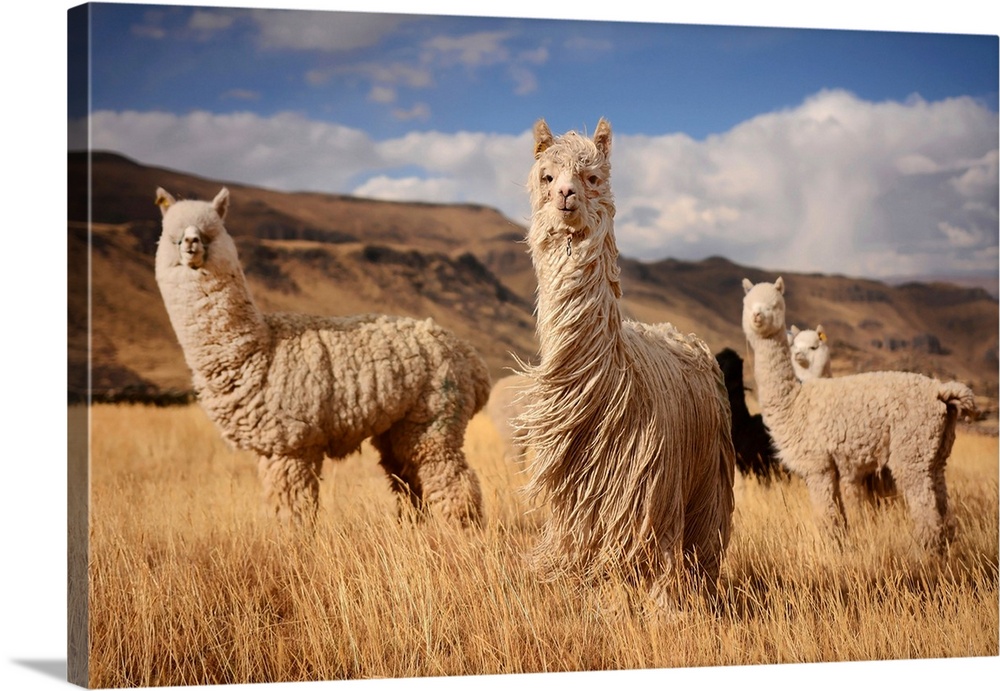The image features a picturesque scene of four llamas, or possibly alpacas, set against a backdrop of barren mountains and a clear blue sky dotted with fluffy white clouds. The focal point is a white, albeit slightly dirty, long-haired llama in the center, gazing directly at the camera with upright ears and a pleasant expression. Flanking this central figure are two other llamas with shorter, woolly fur, their bodies angled sideways but their heads turned to face the viewer, mirroring the central llama's attentive stance. Partially obscured behind the llama on the right is a fourth llama, only its head visible. This picturesque ensemble stands amidst a field of tall, dried grass, suggesting a fall or winter setting. The photo, printed on a 3D canvas, extends around the edges of the frame, capturing the whimsical and serene essence of these fluffy creatures.